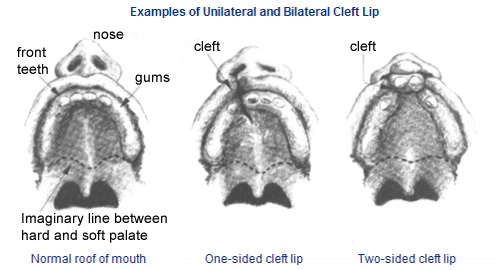The image features a white background with a landscape layout, with the top and bottom longer than the sides. Centered at the top in blue text is the title "Examples of Unilateral and Bilateral Cleft Lip." At the bottom, three detailed digital images are displayed in the center, focusing on the inside of a mouth as if viewed from the chin up, allowing a view of the nostrils and inner mouth structures. 

The image on the left is annotated with black arrows and text explaining the front teeth, nose, gums, and the imaginary line between the hard and soft palate. Underneath it, the blue text reads "Normal Roof of Mouth." The middle image, labeled "One-Sided Cleft Lip," features a line indicating the cleft, displaying a division on the left side of the lip and palate. The right image is marked "Two-Sided Cleft Lip" and shows lines indicating divisions on both sides of the lip, palate, gums, and front teeth. These black-on-white images serve as the focal point, clearly illustrating the differences between a normal mouth and those with unilateral and bilateral cleft lips.